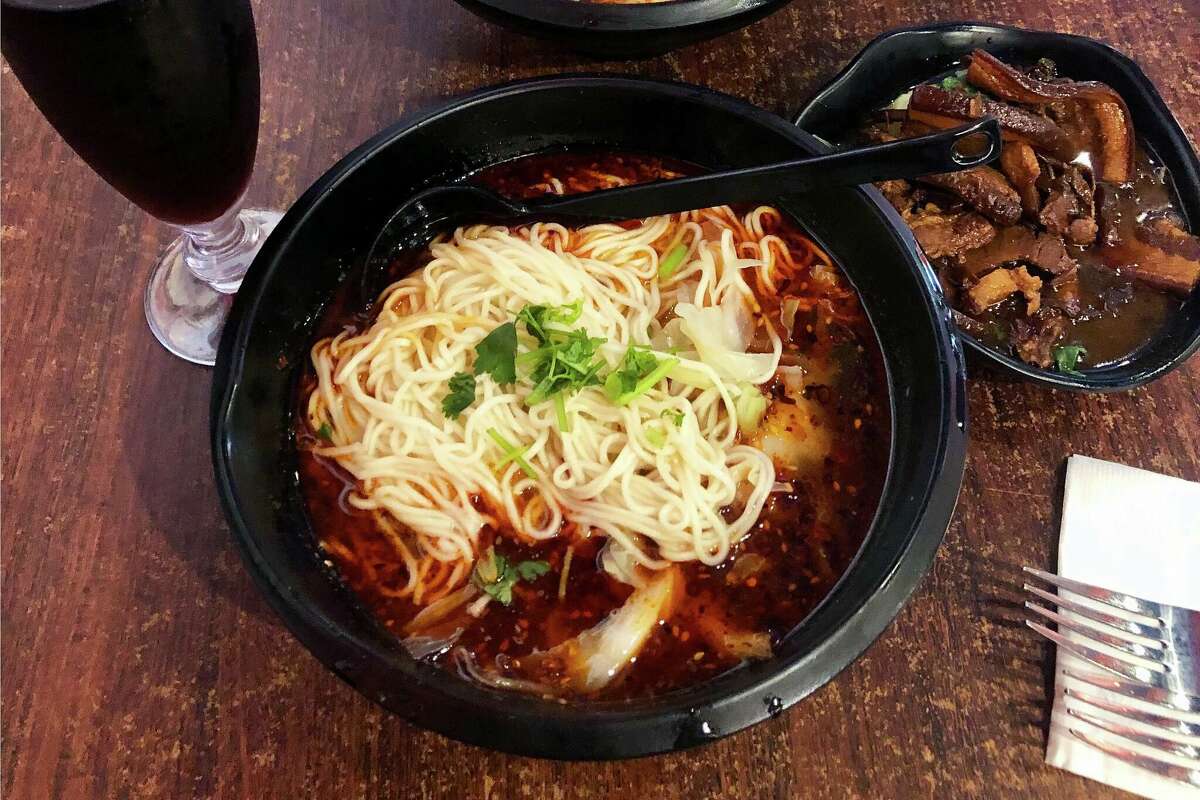The image depicts a detailed scene of a meal set on a dark brown, slightly worn wooden table with visible vertical grain patterns. Central to the image is a large, deep black bowl, likely plastic and possibly disposable, containing a steaming serving of ramen. The ramen consists of thin, white noodles gently curled and clumped together in a vibrant reddish broth that looks spicy, possibly enhanced with red pepper flakes and red pepper oil. Floating in the broth are pieces of vegetables such as cabbage or onion, along with chopped green herbs that could be cilantro or parsley. 

To the upper right of the noodle bowl is a smaller black dish containing pieces of brownish meat bathed in a rich brown sauce, with a sprinkling of herbs but no visible vegetables. The meal is accompanied by utensils: a black plastic spoon rests in the noodle bowl, and a napkin with two forks lies in the lower right corner of the image. To the upper left is a dark beverage in a wine or champagne-style glass, the contents of which could be red wine or a dark soda, adding an elegant touch to the setting. The light source, coming from the lower right, highlights parts of the bowls and adds a warm ambiance to the meal presentation.